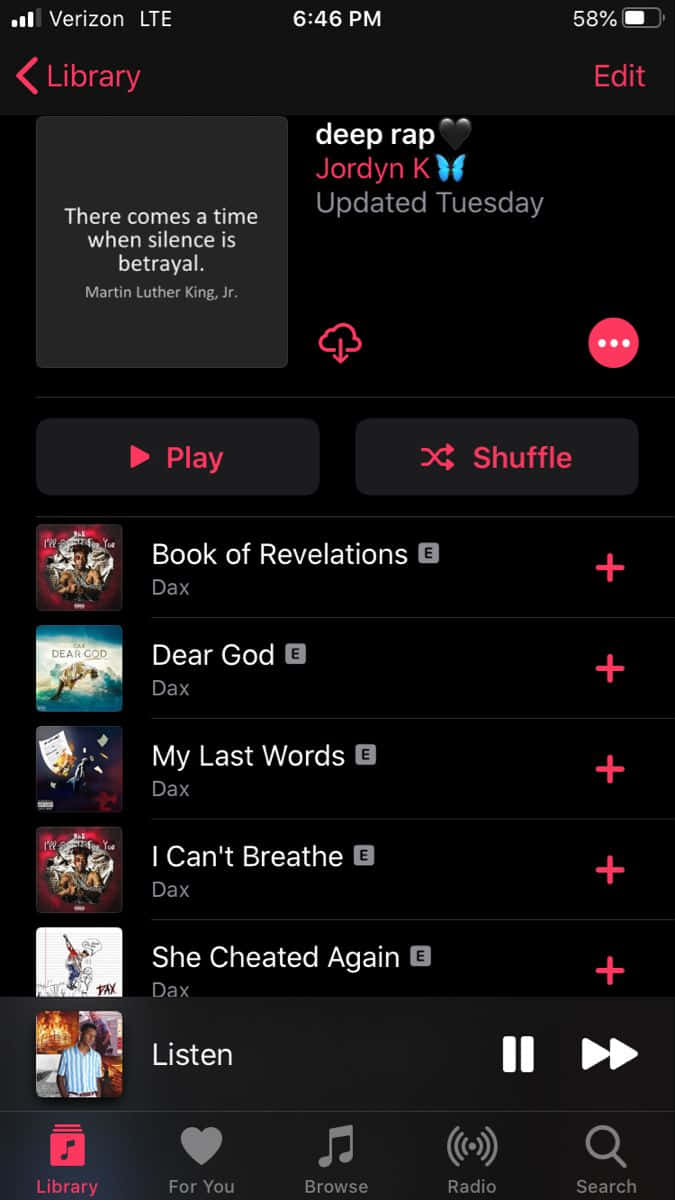This screenshot displays the interface of a music or audiobook application set against a black background, captured from a cell phone screen. 

### Top Section:
- **Notification Bar:**
  - **Left:** Three white Wi-Fi bars.
  - **Center:** The carrier is displayed as "Verizon LTE," and the time is shown as 6:46 p.m.
  - **Right:** Battery status is at 58%, represented by a battery icon with a white fill and a gray outline.

- **App Navigation:**
  - **Top Left:** A red back arrow.
  - **Center**: The word "Library" in red.
  - **Top Right:** The word "Edit" in red.

### Main Content Section:
- **Quotes:**
  - **Left Square:** Contains a quote in white text: "There comes a time when silence is betrayal" - Martin Luther King Jr.
  - **Right Square:**
    - **Top Text:** "Deep Wrap" in white.
    - **Author:** "Jordan K" in red.
    - **Icon:** A blue butterfly to the right of "Jordan K".
    - **Update Info:** "Updated Tuesday" below the blue butterfly.
    - **Icons:** 
      - **Lower Left Corner:** A red cloud with a downward arrow for download.
      - **Lower Right Corner:** A red circle containing three horizontal white dots.

### Buttons:
- **Left Button:**
  - **Appearance:** Black background.
  - **Icon:** Red right-facing triangle.
  - **Text:** "Play" in white to the right of the triangle.
- **Right Button:**
  - **Icon:** Red shuffle icon.
  - **Text:** "Shuffle" in red to the right of the icon.

### Track or Book Listings:
1. **Book of Revelations** by Dax
   - **Icon:** Red plus sign on the right.
2. **Dear God** by Dax
   - **Icon:** Red plus sign on the right.
3. **My Last Words** by Dax
   - **Icon:** Red plus sign on the right.
4. **I Can't Breathe** by Dax
   - **Icon:** Red plus sign on the right.
5. **She Cheated Again** by Dax
   - **Icon:** Red plus sign on the right.
6. **Listen** (No author specified)
   - **Icon:** Young man image in a black, blue, and white striped shirt.
   - **Controls:** Dual vertical pause button lines and two triangle fast forward lines on the right.

### Bottom Navigation Bar:
- **Library:** Red folder icon with a music note next to "Library".
- **For You:** Gray heart icon next to "For You".
- **Browse:** Gray music notes icon next to "Browse".
- **Radio:** Gray soundwave icon next to "Radio".
- **Search:** Gray magnifying glass icon next to "Search". 

This detailed description arranges each element clearly, allowing the reader to visualize the layout and features of the application's interface.